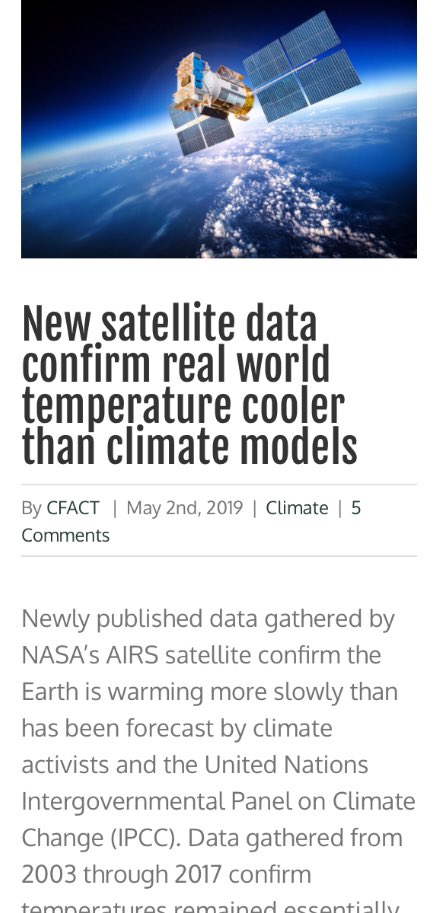This screenshot captures content from an online article viewed on a mobile device. At the top, there's an image depicting a satellite in orbit around Earth, symbolizing the theme of space and climate observation. The layout, characterized by its narrow text arrangement, indicates a mobile screen format.

Below the satellite image, the article's headline reads, "New satellite data confirm real-world temperature cooler than climate models," suggesting that recent satellite data reveal discrepancies between actual temperatures and those forecasted by climate models. 

Following the headline, there is a byline that details the publication date, the author's name, and the total number of comments, providing context about the article's recency and engagement level. The visible portion of the article begins immediately after, though only the first paragraph is shown, hinting at the presence of further detailed content beyond the screenshot's scope.